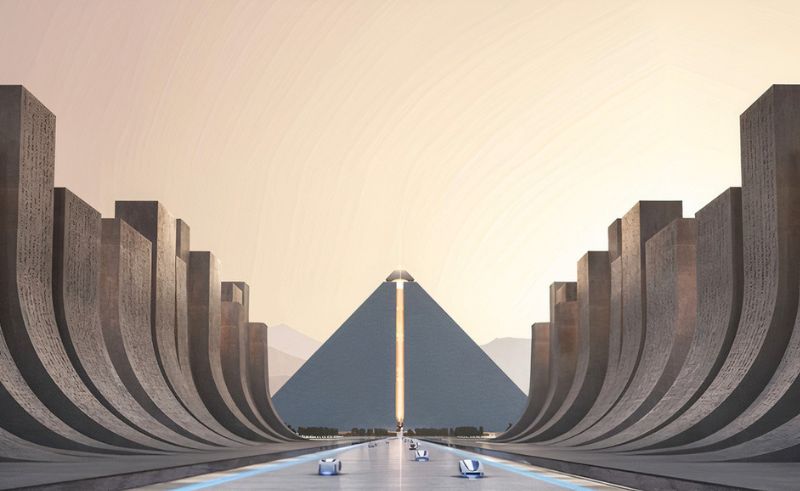The image depicts a futuristic, computer-generated scene with a striking skyline dominated by a light yellow sky featuring concentric circles emanating from a bright source of light. The focal point is a tall, black triangular structure resembling a pyramid, with an opening at its center through which a bright light beam ascends toward the sky, creating a striking visual effect. Surrounding the pyramid, the scene includes a smooth, reflective silver roadway extending towards the structure, populated by several small, shiny objects that resemble futuristic vehicles or robots in silver, blue, and white hues.

Flanking this central roadway on both sides are gently curved, light brown walls of varying heights, creating a wave-like pattern that adds to the modern, otherworldly aesthetic. These walls are not identical on both sides but share a similar design language. In front of the pyramid, appearing to be closer to the viewer, there are sections of walls or possibly hedges, adding layers to the scene's depth. The landscape is devoid of any living beings, enhancing the surreal and serene atmosphere of the image. The overall palette of browns, yellows, whites, blues, and silvers contributes to the high-tech yet tranquil ambiance of the scene.